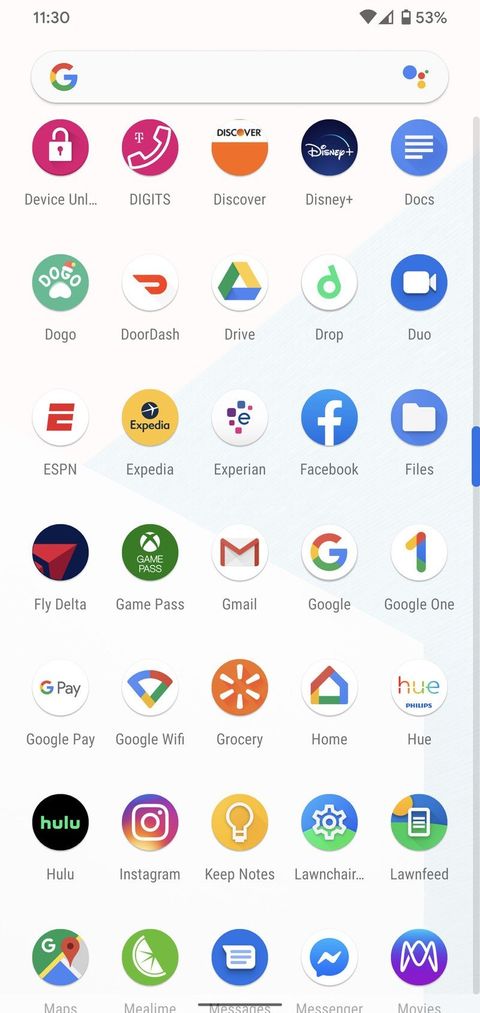The image showcases the home screen of a smartphone, displaying multiple rows of app icons. At the top of the screen, the time is displayed as 11:30 AM, and the battery life indicator shows 53%. Below this, there is a Google search bar with the "G" logo, accompanied by blue, red, yellow, and green accents, indicative of the Google Assistant feature.

The home screen consists of a total of seven rows, each containing five app icons. At the top row, there is a device management app labeled "CUNY" featuring a pink lock icon. The other apps in this row include Digits with a phone icon, Discover, Disney Plus, and Google Docs.

The following rows contain a variety of popular apps, organized as follows:
- Second Row: Adogo, DoorDash, Google Drive, Dropbox, Google Duo.
- Third Row: ESPN, Expedia, Experian, Facebook, and Google Files.
- Fourth Row: FlyData, X Games, Gamerfest, Gmail, Google, and Google One.
- Fifth Row: Google Pay, Google Wi-Fi, Grocery, Google Home, and Hue.
- Sixth Row: Hulu, Instagram, Keep Notes, Lawn Chair, and Lawn Feed.
- Seventh Row: Google Maps, Mealtime (featuring a lime wedge icon), Messages, Facebook Messenger, and Google Movies.

This detailed organization allows easy access to a diverse range of applications, covering everything from social media and entertainment to productivity and financial tools. The screen's layout indicates the user's preference for a structured and well-organized interface.